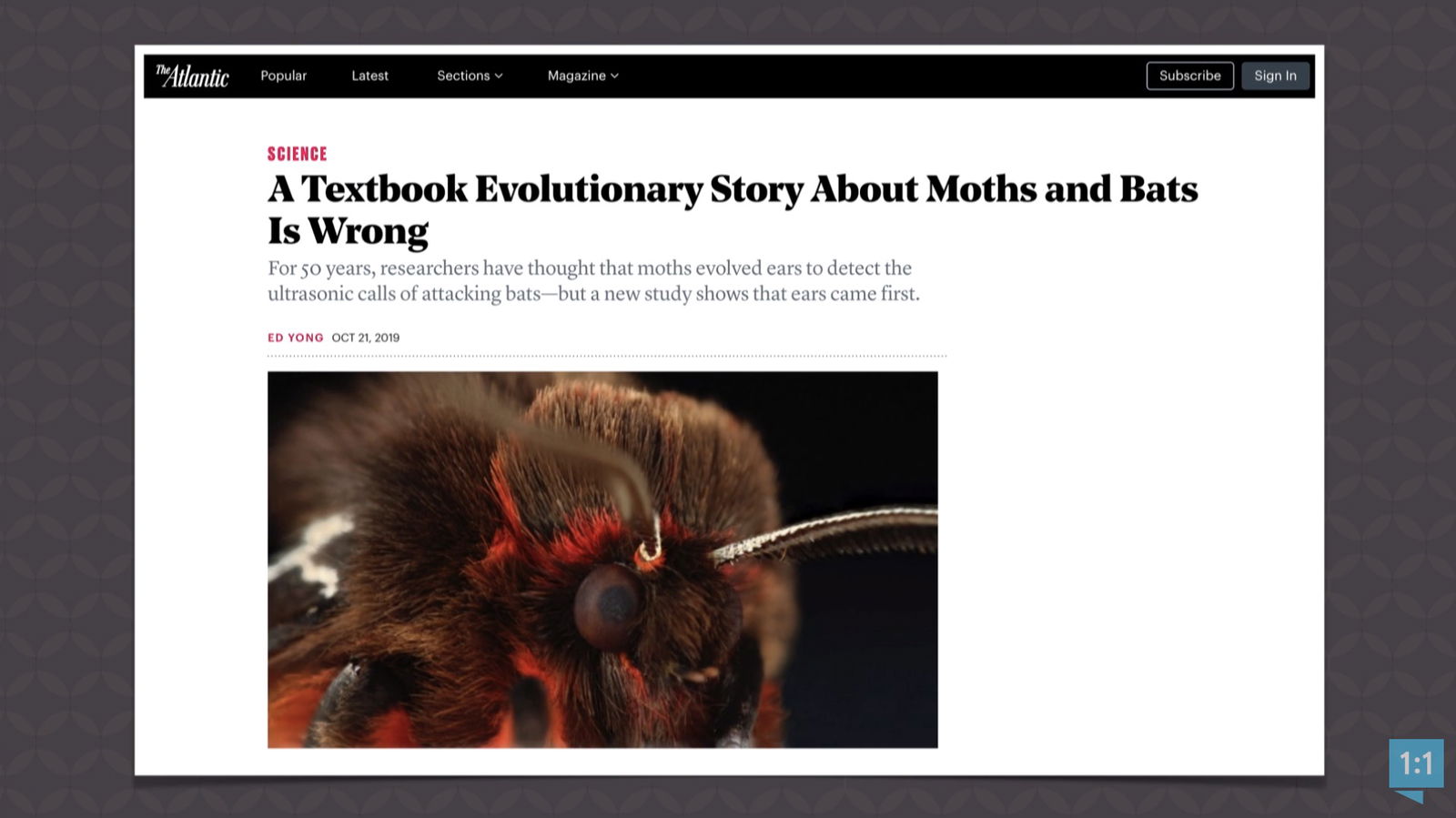This is a detailed descriptive caption for the image of The Atlantic's website:

"The Atlantic's website showcases a sleek black navigation bar at the top featuring section headings in white font, which are clickable for easy access. On the left side, the site prominently displays 'The Atlantic' logo followed by navigational links labeled 'Popular', 'Latest', 'Sections' (with a drop-down menu), and 'Magazine' (with a drop-down menu). Positioned to the right, the site offers options to 'Subscribe' and 'Sign In'.

Below the navigation bar, the main content area highlights an article headline in bold, capitalized pink font: 'SCIENCE'. Directly beneath this, in larger black font, the article title reads: 'A textbook evolutionary story about moths and bats is wrong.' A brief summary follows in smaller font: 'For 50 years, researchers have thought that moths evolved ears to detect ultrasonic calls of attacking bats. But a new study shows that ears came first.' The article is authored by Ed Yong and is marked with a timestamp: October 25, 2019. At the bottom of the page, there is an accompanying image of a moth, relevant to the article's content."